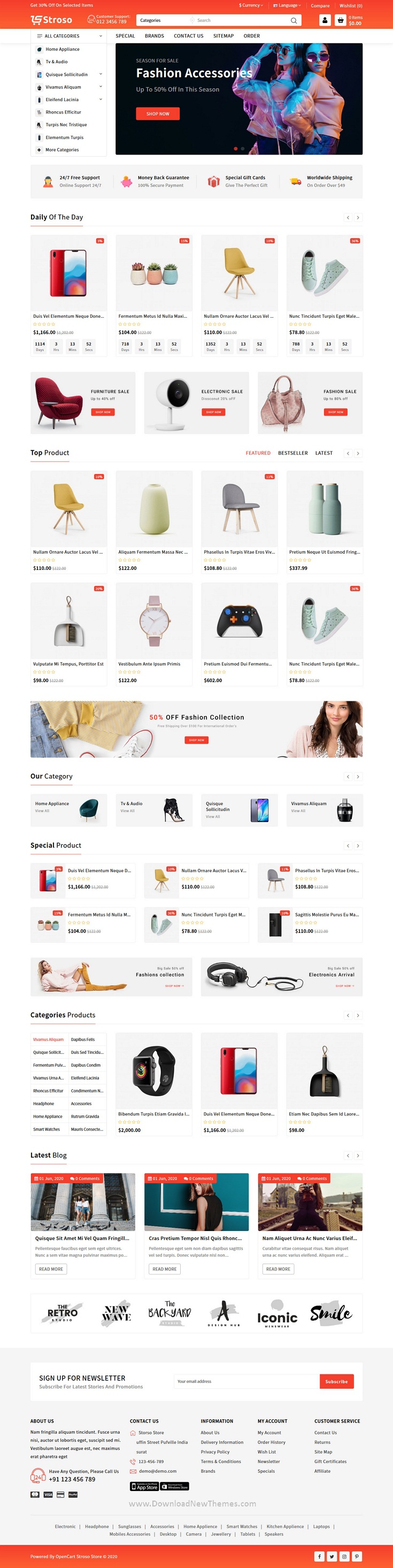The image portrays an extensive, scrolling webpage from an online shopping store, filled with various product listings. Each item is depicted with a distinct icon, though the details appear quite small. Among the array of items, notable products include a phone, a yellow chair, a single maroon chair or couch, a handbag, a pair of sneakers, candles, bottles, a wristwatch, and a PlayStation console. The page is densely populated, featuring a multitude of diverse items, showcasing the variety available in this online store.